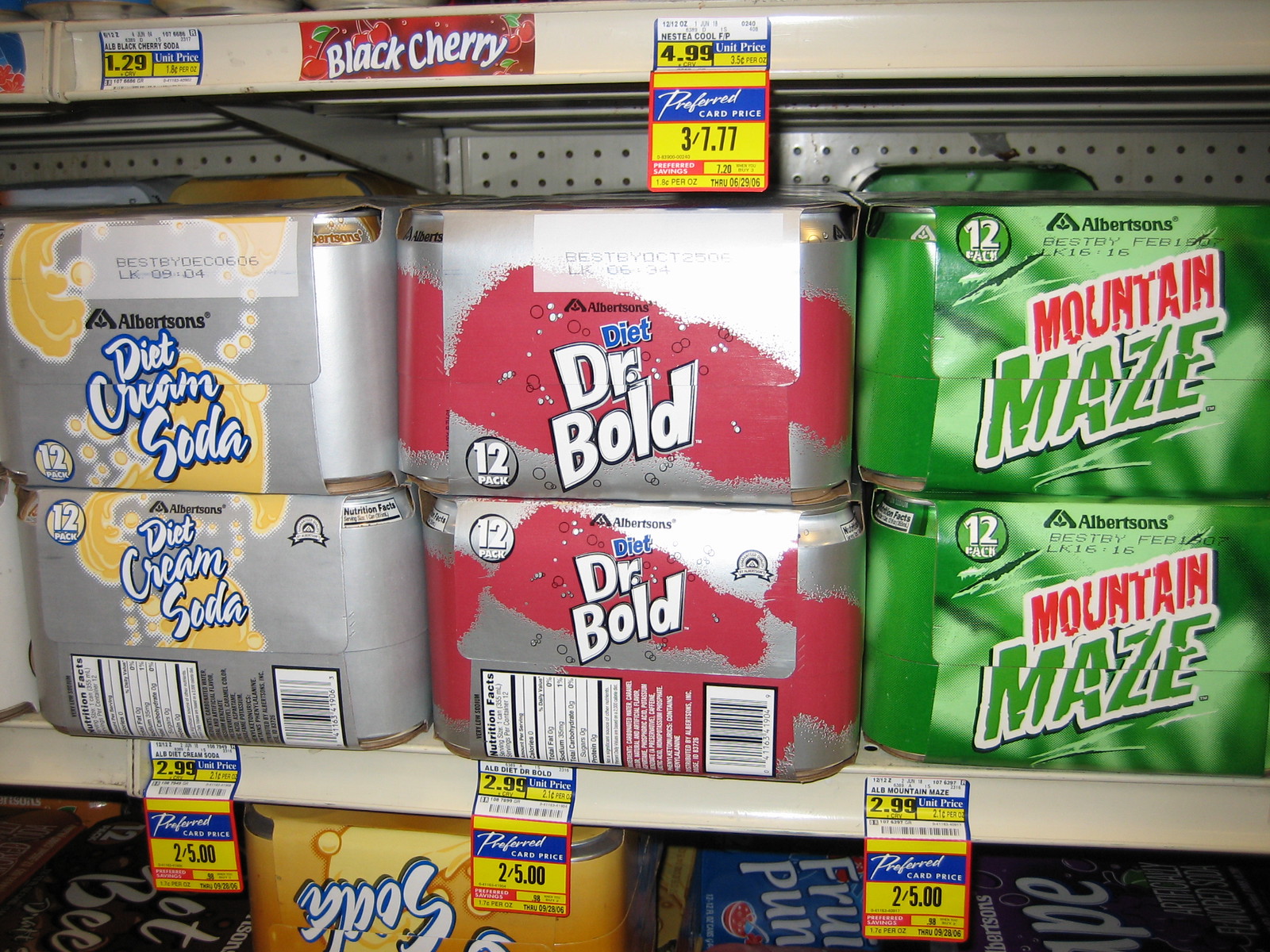The photograph captures well-organized supermarket shelves inside an Albertsons grocery store, evident from the readable product names on the labels. The image focuses on two shelves adorned with vibrant price tags in hues of blue, yellow, and red. These shelves prominently display an assortment of 12-packs of soda. 

On the right side of the shelves, there are two 12-packs of soda in green packaging, distinguished by red "Mountain" lettering and green "Maze" text. In the middle section, slightly to the left, is a stack of two silver packages with striking splashes of red paint. These feature the label 'Diet' in blue and 'Dr. Bold' in white. Moving further to the left, another silver package catches the eye; this one has red splashes and bears the name "Diet Cream Soda" elegantly written in white cursive lettering. The meticulous arrangement and vivid packaging make for a visually appealing and organized display.